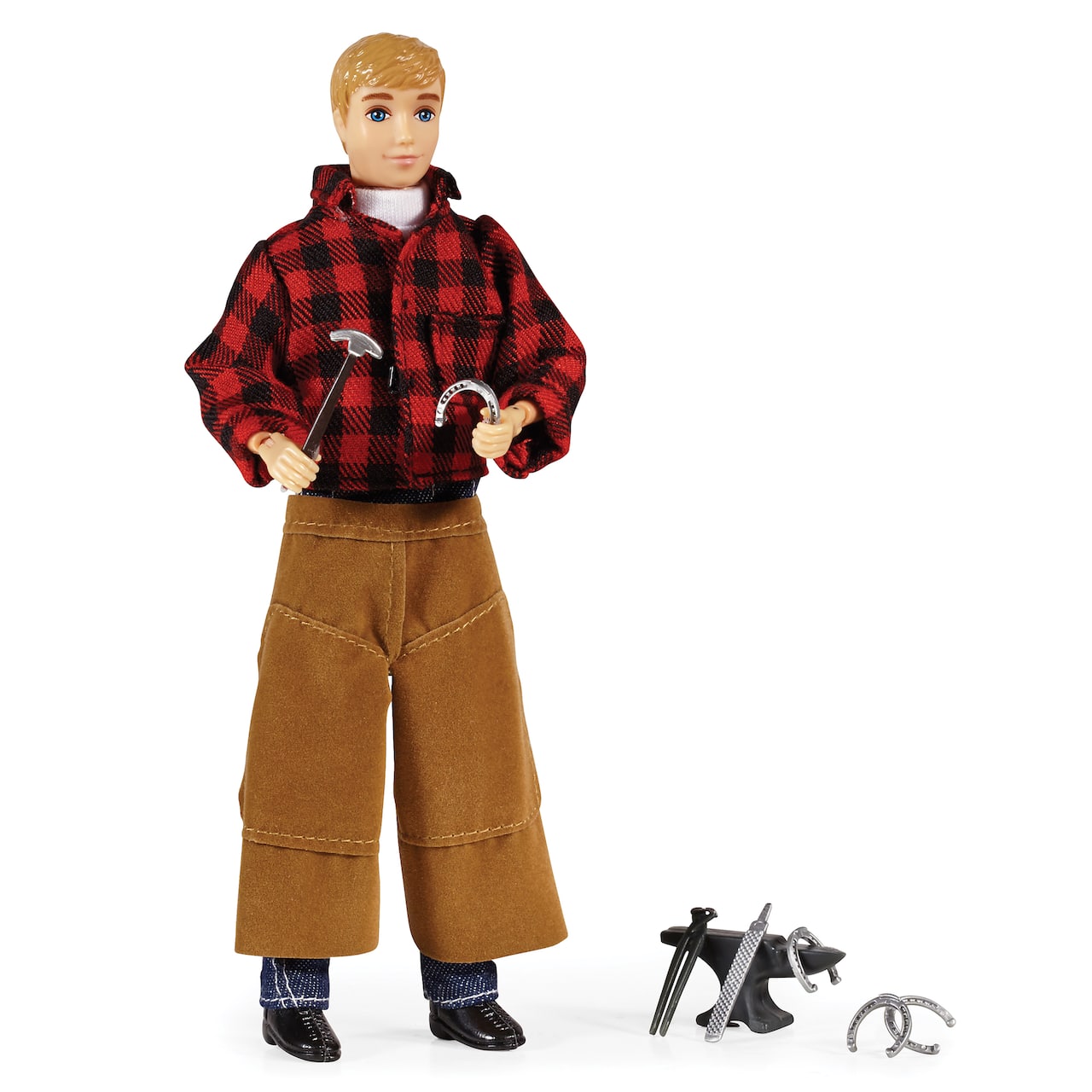This photograph features a male doll resembling a Ken doll, showcasing particular craftsmanship details. The doll has short blonde or light brown hair and striking blue eyes, set against a backdrop of Caucasian skin. Adorning his upper body is a distinctive black, red, and white checkered shirt draped over a white undershirt. He is dressed in brown pants that flare slightly at the bottom, revealing blue jeans underneath. His footwear consists of shiny black shoes. 

The doll is engaged in a blacksmithing scenario, holding a hammer with a black handle and silver head in his right hand, and a horseshoe in his left hand. The scene is further illustrated by various tools scattered on the floor beside him: a black anvil sits with a horseshoe draped over it, accompanied by a file, a pair of pliers, and two additional silver horseshoes. 

Set against a plain white background, this meticulous and imaginative depiction likely represents a blacksmith, emphasizing the doll's crafted appearance and the tools of his trade.